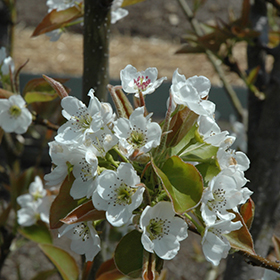A high-resolution, square, outdoor photograph captures a close-up view of a cluster of white flowers in full bloom, which appear to be fruit tree blossoms, possibly apple or crabapple. The flowers, each with five petals and tiny brownish dots in the center, are prominently situated on a thick branch amidst a mix of heavy-duty green leaves. The background is intentionally blurred, creating a bokeh effect that emphasizes the foreground blossoms. In the background, there are visible tree trunks and branches, with light-filtered layers of gray, tan, and green suggesting a sunlit outdoor setting. The image conveys a serene, natural scene likely taken in a park, where the detailed texture and delicate beauty of the blossoming flowers are brought into sharp focus against the muted backdrop of the surrounding trees and foliage.